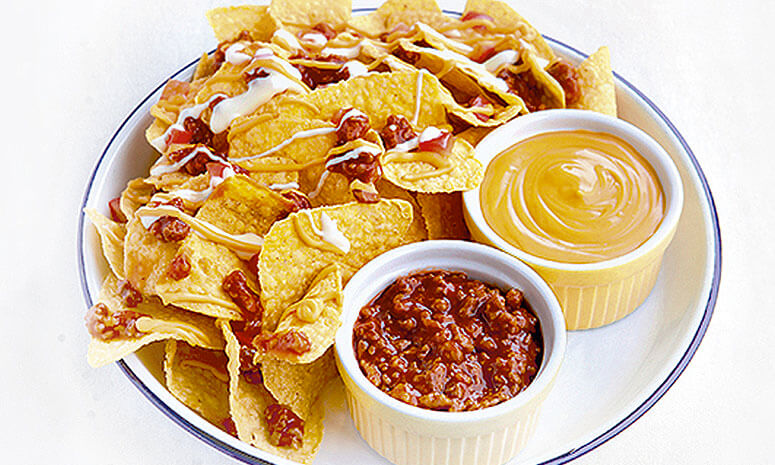The image features a round white plate, possibly made of china, with a distinctive blue trim around the edge. The plate is filled predominantly on the left side with crisp yellow corn nacho chips. These chips are generously drizzled with a blend of pale yellow, orange cheese, and a white sauce that appears to be sour cream. Scattered atop the nachos is a red chili, likely resembling the contents of one of the ramekins. Situated on the bottom right of the plate are two small white glass ramekins; one brimming with a smooth, melted yellow cheese sauce, and the other containing a hearty chili made with ground meat and tomato sauce. The background is a simple, off-white color, drawing focus entirely to the delectable nachos and their flavorful accompaniments. The overall presentation looks delicious and inviting, capturing a close-up, slightly downward-angled view.